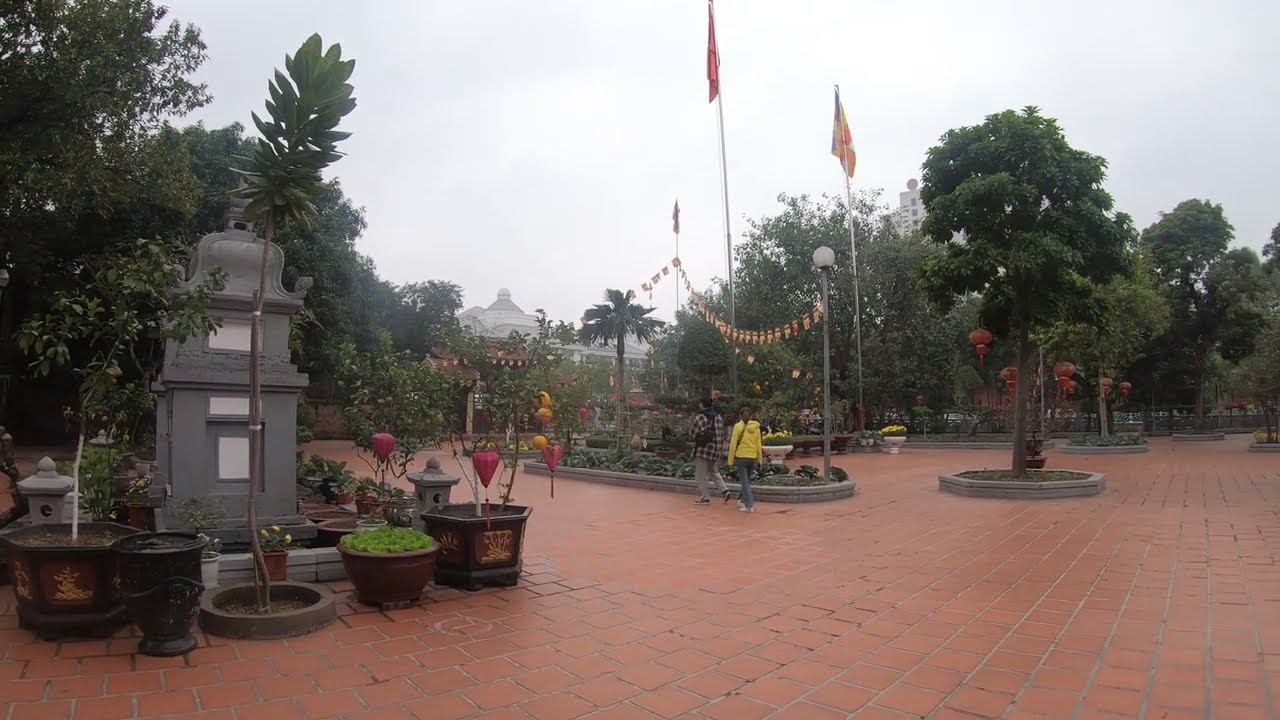The image depicts an expansive outdoor space, reminiscent of a botanical garden or public park, with the ground covered in terracotta-like orange brick tiles held together by gray mortar. Dominating the right side is a large, green-leaved tree with a brown trunk, encircled by a concrete ring. Near the top left of the tree, three flagpoles stand tall, with the tallest pole flying a red flag, while the other two flags are less distinguishable. A banner, seemingly yellow, is strung from light poles and dips gracefully before rising to another pole.

In the foreground, there are people walking in opposite directions along the brick walkway. One individual, wearing a yellow shirt, dark jeans, and a black strap over one shoulder, appears to be of African descent. Trailing behind is another person in a plaid shirt, khaki pants, and also carrying a black bag. 

The background features a large building with a dome that rises above the scene, indicating a historical or significant landmark. On the left, partially obscured by a thin tree with silver rings around its trunk and broad green leaves, is another domed structure. Beneath this tree are several potted plants, mostly in black pots, with one notable brown pot. The brown pot contains plants that have air-filled, heart-shaped objects, possibly made from paper mache, resembling the blossom of a bleeding heart plant. Overall, the scene under a bright, clear sky with vibrant colors, suggests a serene, well-maintained environment, bustling with life and activity.